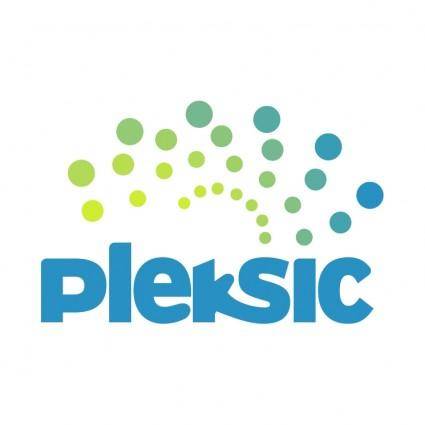The image showcases what appears to be a digitally generated logo, potentially for a company or a product. The prominent text in the logo reads "Plexic" in a bright blue color, with a notable design where the 'K' connects to the 'S'. Above the text, a series of colored circles is arranged in an arch reminiscent of a rainbow. These circles exhibit an ombre effect, transitioning from light green to darker green, and then from bluish-green to darker blue as they move from left to right. The circles also vary in size, being larger at the top of the arch and getting progressively smaller as they approach the word "Plexic." The overall design and vibrant color scheme suggest a modern, digital aesthetic likely created using graphic design software.